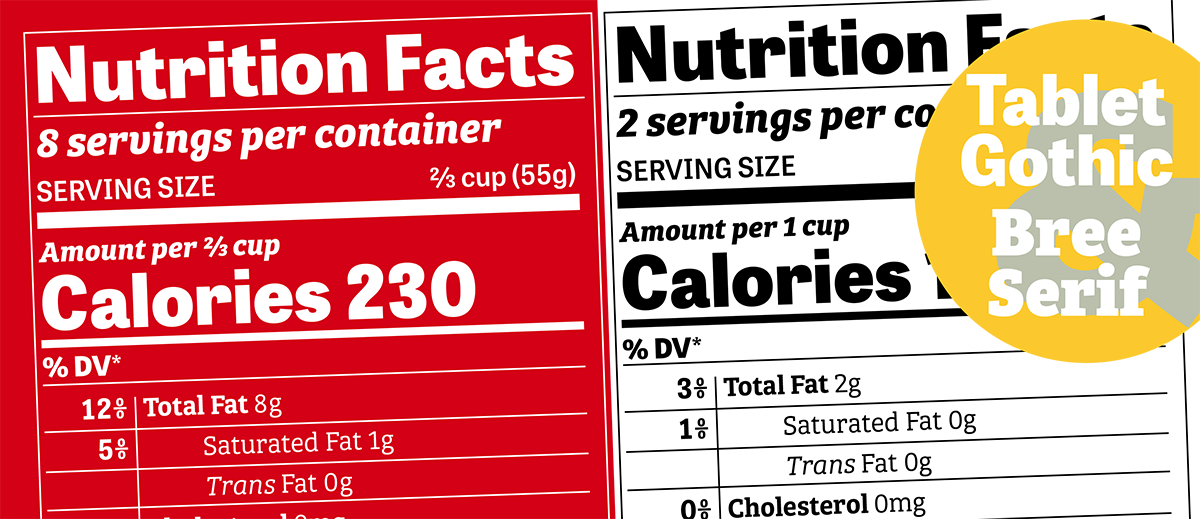This image features a carefully curated compilation of vector graphics primarily showcasing text elements, likely intended as a font sample or advertisement. Dominating the right side of the image is a vibrant yellow circle, centrally adorned with an olive green ampersand symbol. Overlaying this circle in crisp white text is the label "Tablet Gothic Breeze Serif," indicating the font being highlighted.

Positioned behind the yellow circle are dual examples of graphic design implementations using this specific font. The designs illustrate potential uses of the typeface in presenting nutrition facts, akin to those found on food packaging. On the left, the nutrition facts are displayed against a striking red background with white text, creating a bold contrast. Conversely, the right example features a more traditional layout with black text on a pristine white background. Together, these elements provide a comprehensive visual demonstration of the versatility and application of the "Tablet Gothic Breeze Serif" font in various design contexts.